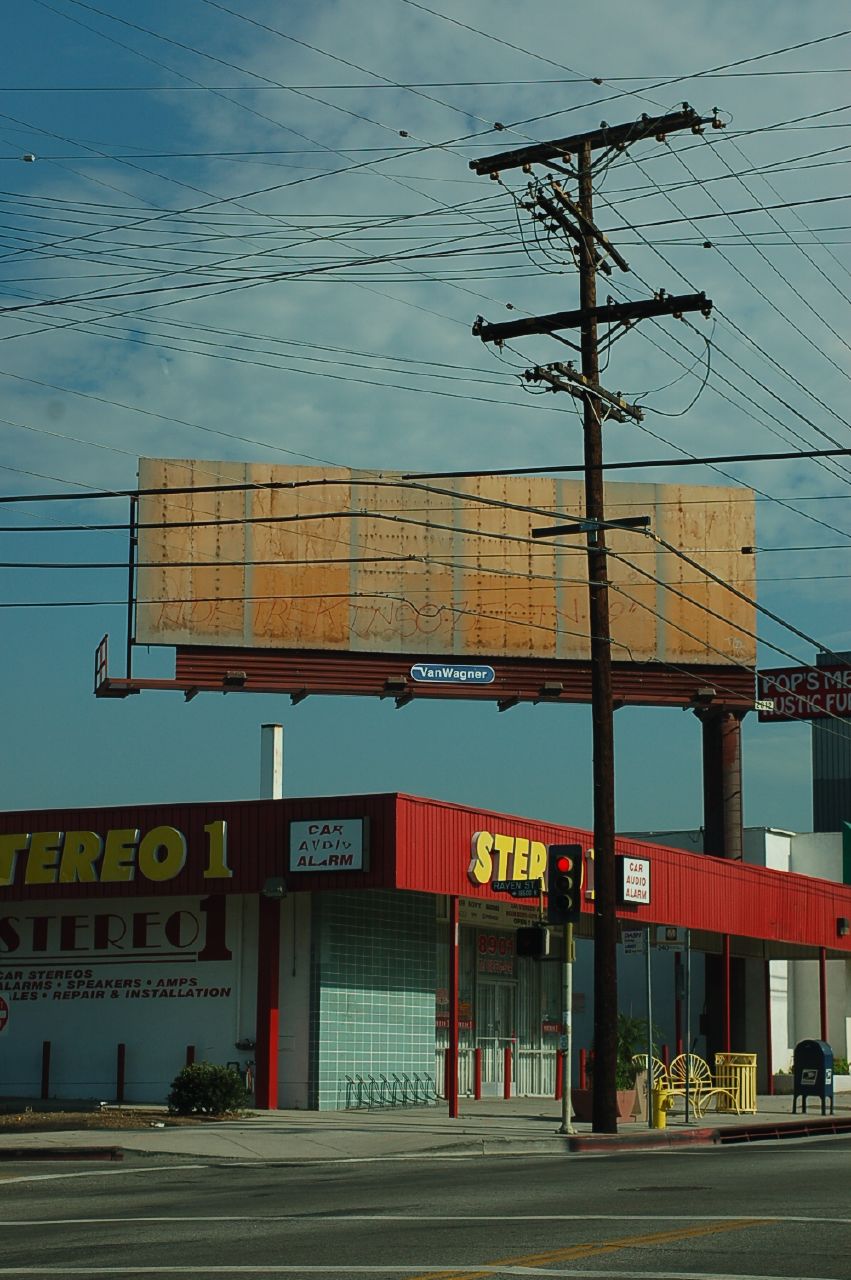The image captures a rundown neighborhood during daytime with a clear blue sky featuring loose, fluffy clouds. Dominating the scene is a red-topped, one-story store named "Stereo One," with its yellow signage clearly displayed. To the left of the store, a red traffic light and a street sign indicating "Raven Street" are visible. The store appears closed and somewhat dilapidated. There's a large, rectangular wooden billboard above the store, which is entirely empty, except for a small piece of text that reads "Van Wagner" with some graffiti. Various yellow street furnishings—including benches, a hydrant, and a garbage can—and a blue mailbox bin dot the sidewalk, adding to the urban clutter. A tall telephone pole with multiple electrical wires stands prominently in front of the store, reinforcing the area’s worn-out appearance.